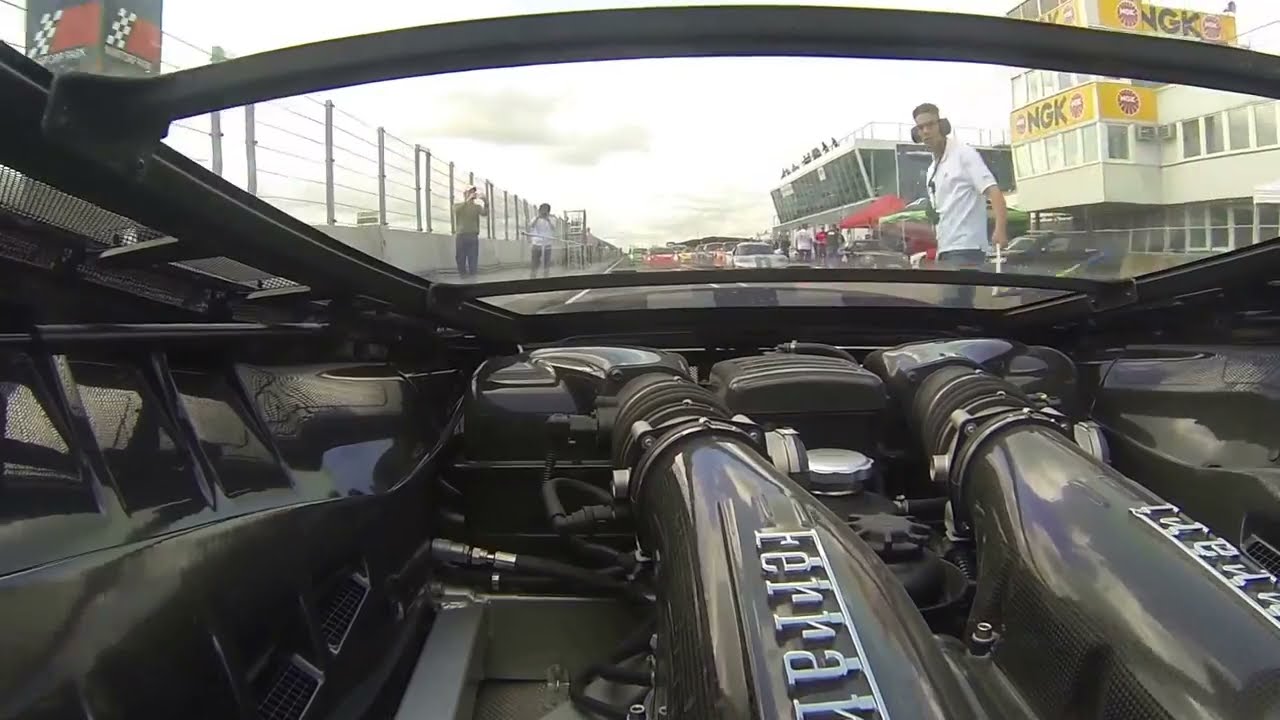The photograph captures a close-up view from the rear window of a Ferrari, specifically focusing on its rear-mounted engine. The shiny black metal components feature a prominently displayed Ferrari logo in silver. The image is taken from an angle where it looks like someone has turned around from the front seat to photograph the inner workings of the car. Beyond the car's glass window, a racetrack comes into view, characterized by various structures including an air traffic control-like tower, spectator boxes labeled with Asian text, and buildings on the left. The scene is busy with contenders, photographers, attendants, and officials, including a person wearing a red and white polo shirt with pants and a headset. Other cars are also visible lined up behind the Ferrari, emphasizing the bustling race-day atmosphere. The vantage point and details together narrate a dynamic scene combining technical automotive craftsmanship with the lively energy of a race event.